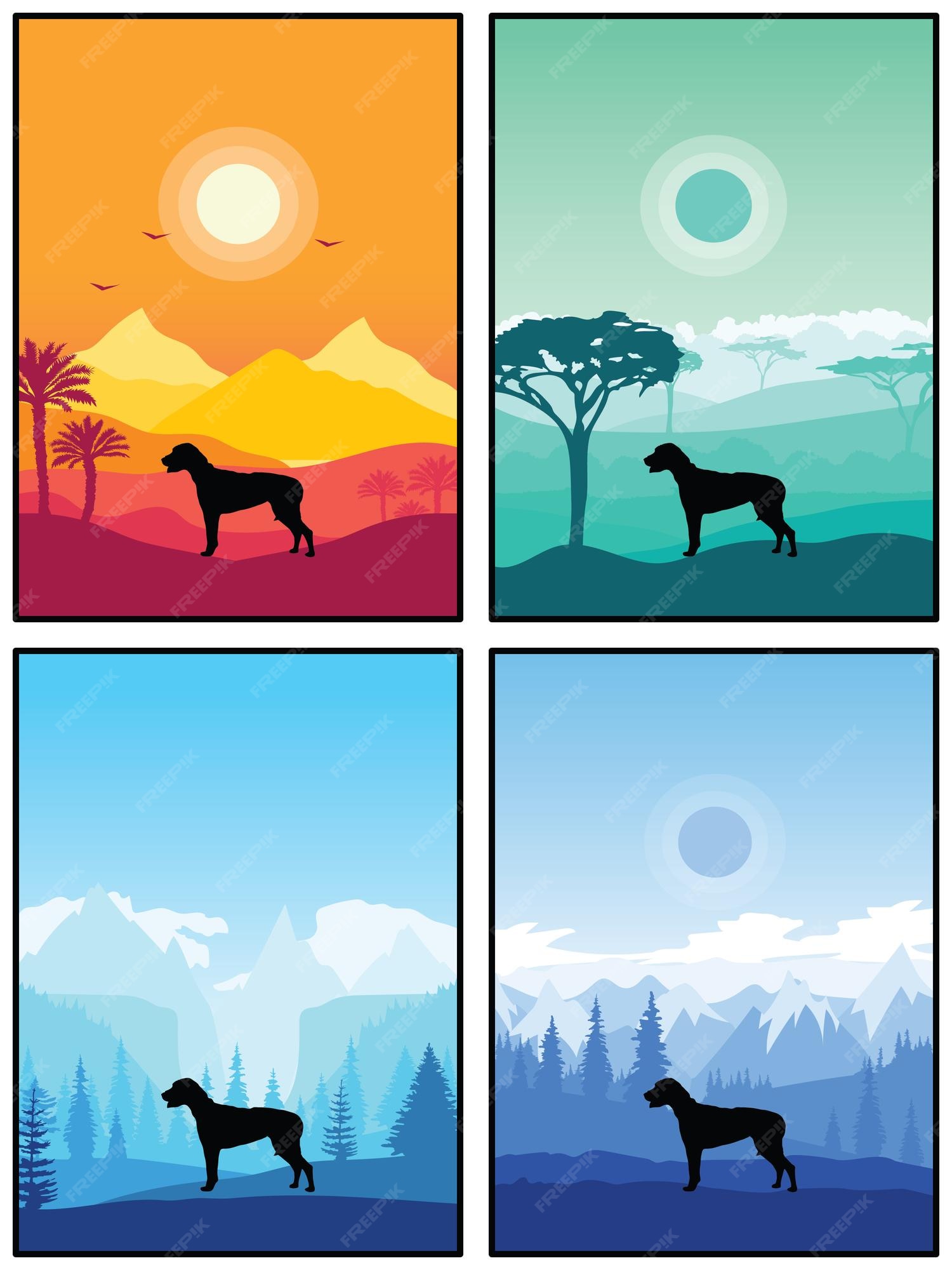The artwork is a vibrant collage consisting of four images, each featuring the silhouetted figure of a dog in the foreground. The images are arranged in two rows of two. 

In the top left image, the dog stands against an orange desert backdrop, illuminated by a bright sun with mountains painted in hues of yellow and orange. Palm trees and red sand add to the warm, arid landscape, and three birds can be seen flying in the background.

The top right image transports the dog to an African setting, characterized by acacia trees. The scene is dominated by green tones, with a light green sky and sand, and a sun tinted in green.

The bottom left image presents a winter scene, where the dog is silhouetted against a backdrop of tall evergreen trees and cliffs. The sky transitions from light blue at the top to dark blue at the bottom, creating a cold, serene atmosphere.

In the bottom right image, the dog remains the focal point in a similar winter setting but with a more intense blue palette. Snow-capped mountains are visible under a darker blue sky, with the sun shining from the same position as in the previous images.

Each panel emphasizes not only the consistent positioning of the dog but also the variation in color palettes and backgrounds, showcasing a range of natural environments.